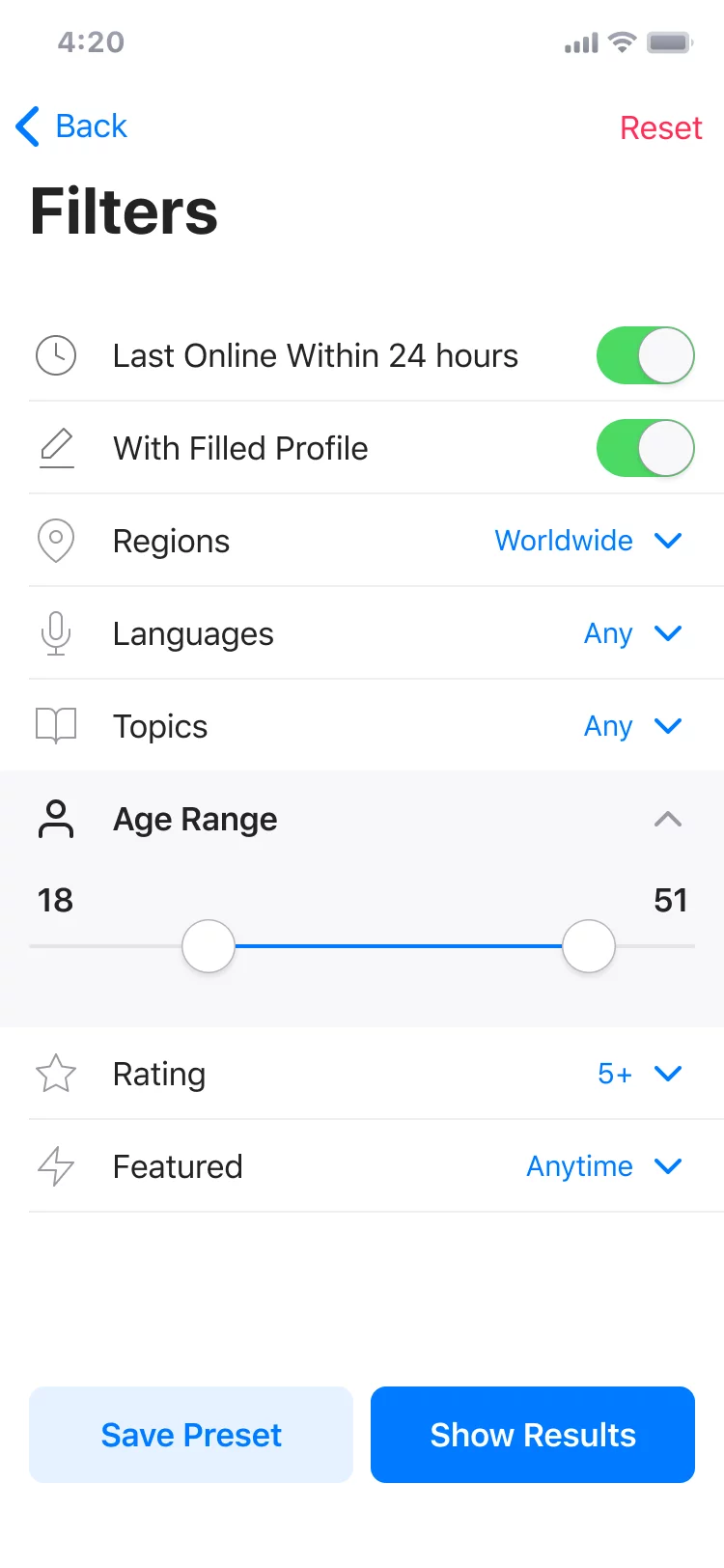### Detailed Caption:

This image captures a smartphone screen displaying a specific interface likely associated with a social or connectivity-based application, categorizing it under "Websites". The time shown at the top of the screen reads 4:20, though it is unclear whether it is AM or PM. This timestamp is displayed in grey lettering at the top of a white background.

Adjacent to the time, on the extreme left, are signal strength bars which indicate full reception. Next to the signal bars is the Wi-Fi symbol, showing that Wi-Fi is enabled, and on the far right of this same header line is the battery icon, indicating a fully charged battery.

Directly beneath this heading, the word “Back” is displayed in blue, accompanied by a clickable arrow for returning to a previous page. Beside it, in red text, the word “Reset” appears, serving as a reset button.

The central portion of the screen features the title “Filters,” followed by several filter settings. These settings include:
- **Last Online:** Within 24 hours (enabled)
- **Profile Filled:** On (enabled)
- **Regions:** Worldwide (with a dropdown arrow, indicating the option to select different regions)
- **Languages:** Any
- **Topics:** Any
- **Age Range:** 18 to 51
- **Rating:** 5+ 
- **Featured:** Anytime

At the bottom of this section, there are options to either “Save Preset” or “Show Results.” The overall appearance and specifics of the filters suggest that it might be an application intended for social interaction, possibly for connecting with pen pals or forming online friendships, rather than a conventional dating app.